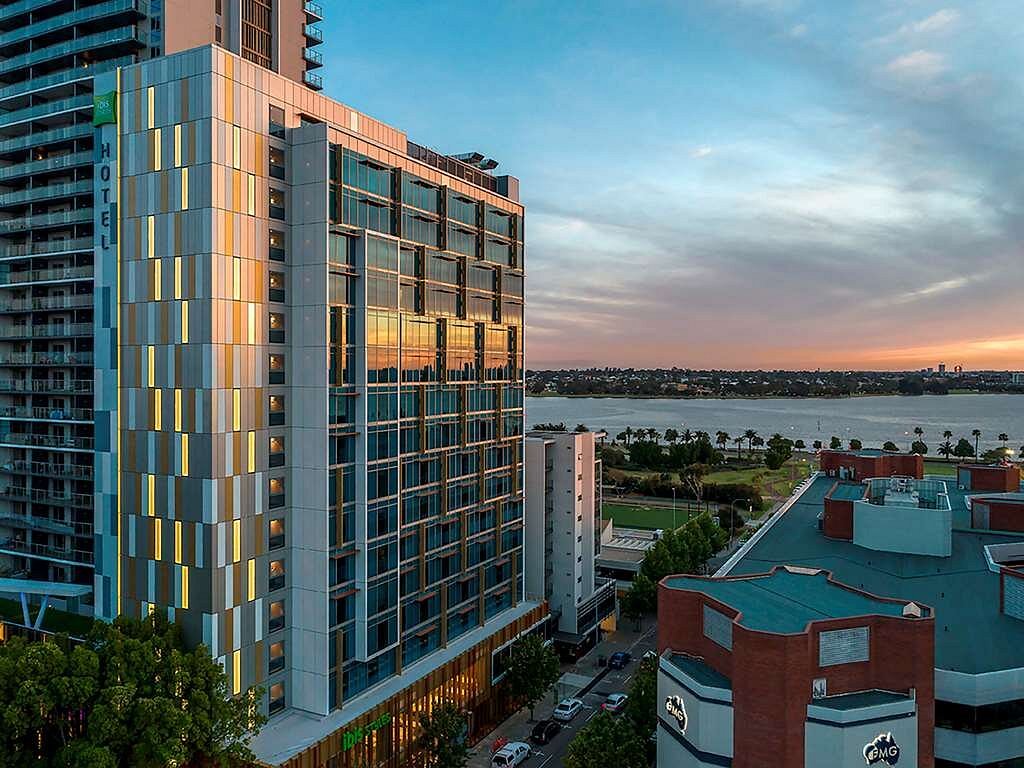A scenic photo captures a striking modern hotel, prominently featuring large glass plate windows, possibly taken from an elevated vantage point or a drone. The building has a unique, late 70s architectural style, accented by colorful blocks in varying shades of pink, orange, gray, black, blue, light blue, and white, forming a vibrant contrast against its contemporary elements. Adjacent to this hotel, there is a smaller, gray building with maroon posts, marked with "9MG," further emphasizing the eclectic nature of the scene. The background unfolds into a picturesque harbor lined with numerous palm trees, which suggests a coastal location, likely in Florida or California. The waterway, flanked by industrial structures and numerous buildings, gleams under the setting sun, casting a serene orange hue across the partly blue sky, enhancing the tranquil yet bustling atmosphere of this urban coastal expanse.